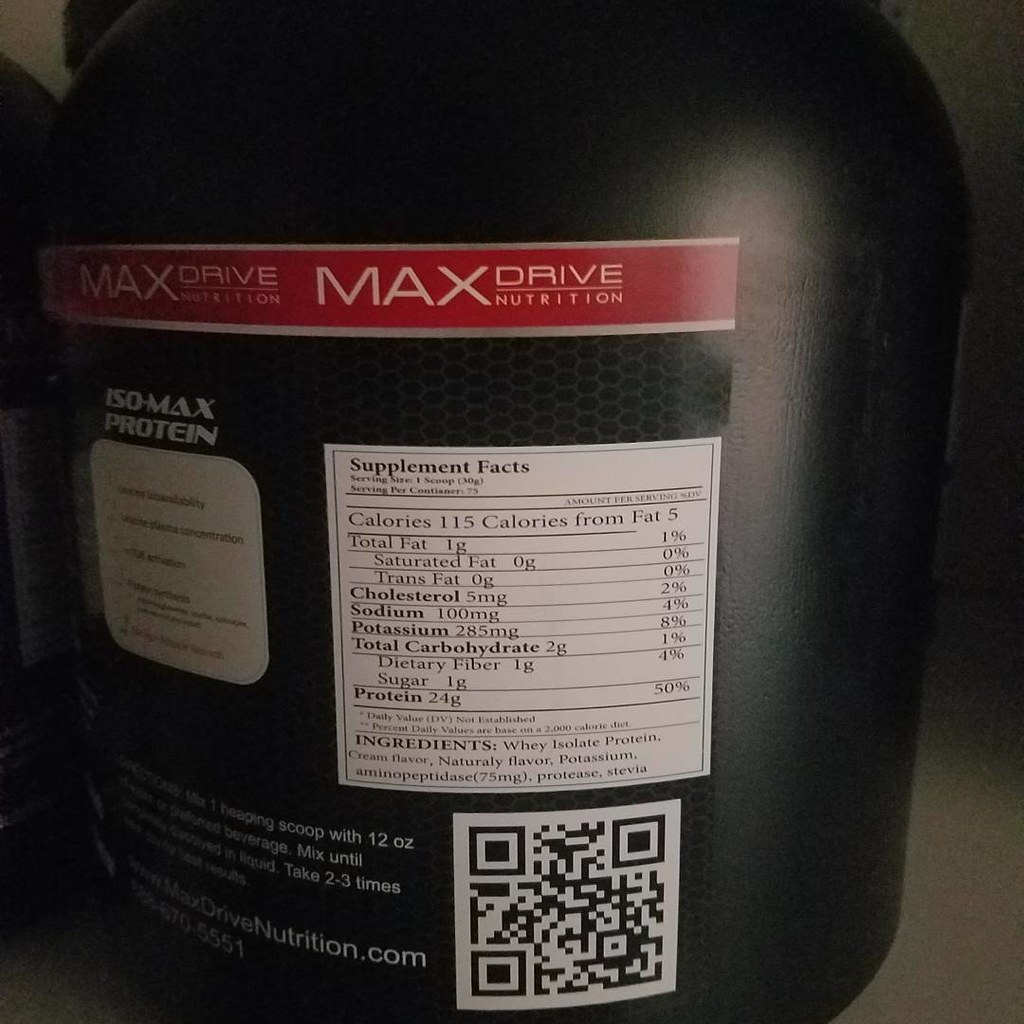The image features the back of a large, black, plastic container of a protein supplement. The label on the container is predominantly red and white. At the top of the label, "Max Drive Nutrition" is prominently displayed in bold, red letters. Directly beneath this, the product name "Isomax Protein" is written, indicating that this is indeed a protein powder supplement.

To the right side of the label, the "Supplement Facts" section is clearly visible. This section provides comprehensive nutritional information about the contents of the protein supplement, detailing various nutrients and their quantities per serving. Beneath this nutritional information, there is a QR code, which likely leads to additional product details or a website for further information.